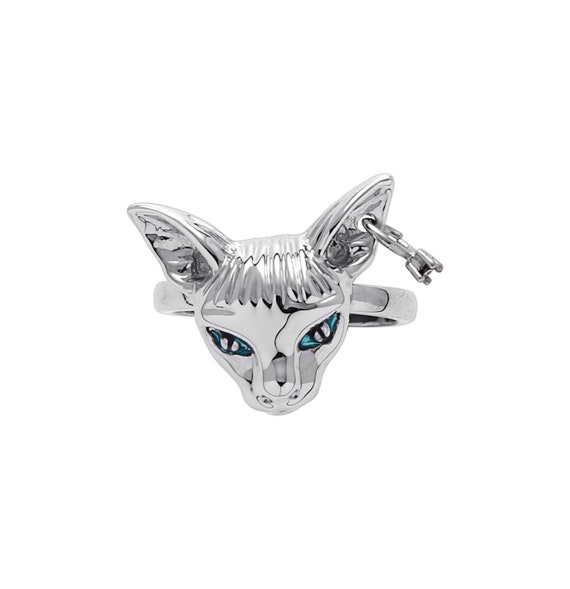This image depicts a silver-colored ring featuring an intricately detailed animal head, possibly that of a cat or a horse, though the exact animal is ambiguous. The head, which could resemble either a sphinx cat or a domesticated animal, stands out with its long, fringe-like hair at the front and large, piercing turquoise blue eyes that seem to change color partway, transitioning to a silvery hue in the middle. The animal's ears are prominent, one of which is adorned with a swivel hook or chain piercing through a hole. The entire composition, including the animal's head and the ring band, is made of metal, sitting on a metallic base that supports the head. The striking features, particularly the intense anime-like eyes and the detailed ear piercing, make this piece notably unique and visually captivating.